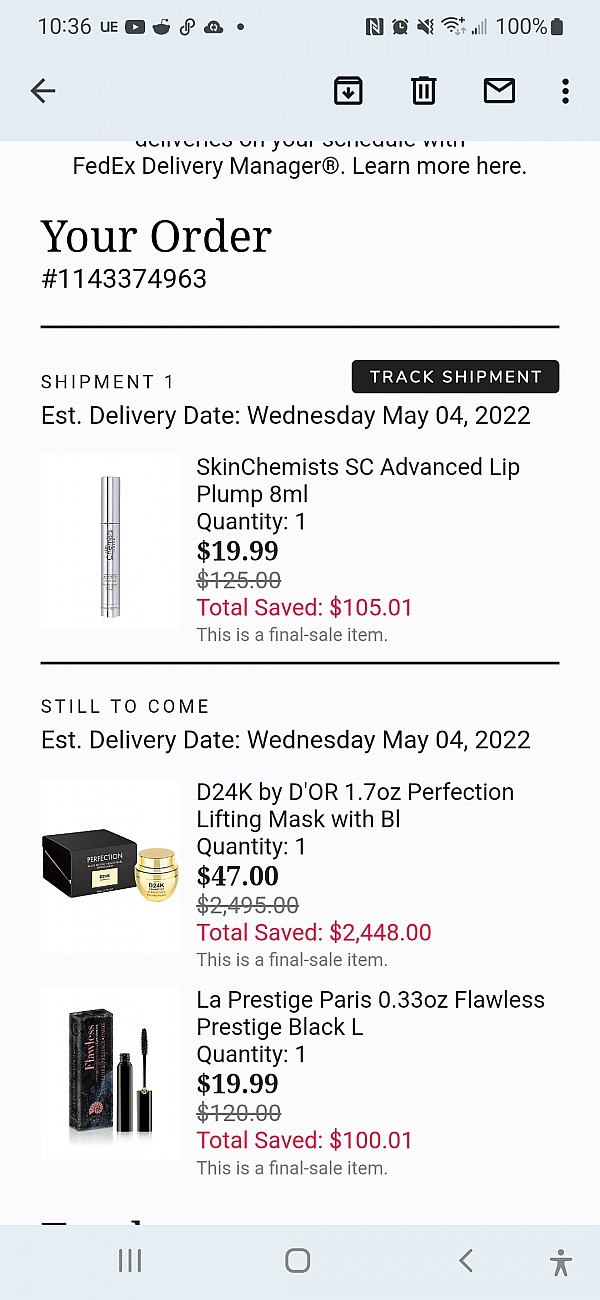This detailed caption captures the essential details vividly for the image described.

---

"Screenshot of an Android phone displaying a website where the user is browsing beauty products. The current time, 10:36, is visible at the top left along with several push notification icons, including Reddit and YouTube. The top right shows the phone's status with a 100% battery life and active data and cell signal connection. 

The website displayed on the screen has a white background and features the user's recent purchases along with their shipping information. The top of the screen prominently displays 'Your Order' in large black text, followed by the order number in smaller text. 

The center of the screen lists three items that the user has purchased: a Skin Chemist SC Advanced Lip Pump (8ml), D24K by Dior Perfection Lifting Mask with BL (1.7oz), and La Prestige Paris Flawless Prestige Black L (0.33oz). Each item includes details about the price, savings, and expected delivery date. 

At the bottom of the image, Android navigation icons - including the back button - are visible, providing the user with options for navigating through their phone."